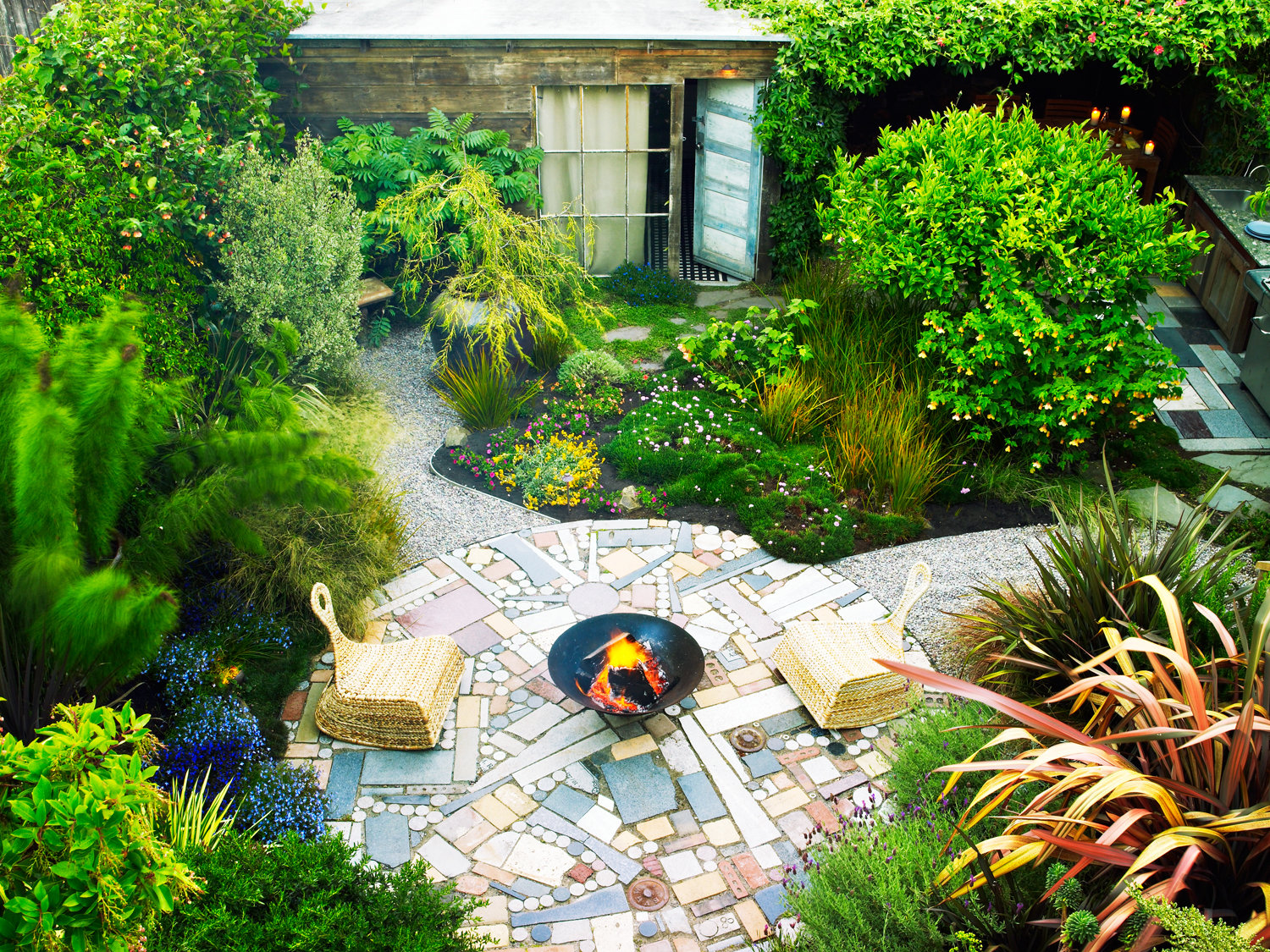This is an overhead view of a beautifully designed backyard featuring a small outdoor bungalow or pool house. The structure is box-shaped and adorned with wood paneling on its front. It includes nine windows, a very large window next to a wooden door painted white and blue, and the front area reveals a large white and black rug through the open door. Surrounding the bungalow is lush landscaping, with numerous plants and trees adding to the serene ambiance. 

In the foreground, there is a circular area made of different colored and patterned stones arranged artistically, surrounded by a gravel walkway. The centerpiece is a black round fire pit with a burning red and orange fire, flanked by two sculptural wicker chairs resembling paintbrushes, characterized by their thin and narrow backs. The gravel walkway extends beyond this circular area, leading to various parts of the garden, including a separate gravel trail that winds through the garden and exits the backyard.

Additionally, a glimpse of an outdoor kitchen with a tiled floor in blues and browns can be seen at the top right, further enhancing the space's functionality and appeal. The photograph captures the lush greenery, including several tall trees and flowering plants, some of which display blue blooms at the bottom left corner. This peaceful and stylish backyard invites relaxation and offers a perfect spot for gatherings, with no people captured in this vibrant color photograph.